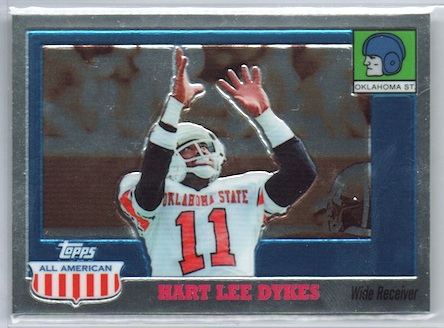This Topps brand All-American sports card, securely housed in a protective covering, features Hartley Dykes, a wide receiver for Oklahoma State. The card showcases a detailed layout with multiple borders: an outer silver frame followed by gray and blue borders, framing the central image. In the center, a black man wearing a white Oklahoma State football jersey with the red number 11 stands with both hands extended upwards as if prepared to catch a pass. He is dressed in black long sleeves and a white helmet. The top right corner of the card has a square with an illustration of a football player wearing an Oklahoma State helmet. The Topps logo, accompanied by a red and white All-American badge, is positioned in the lower left corner. Just to the right of Hartley Dykes’ name, displayed in red capital letters beneath the image, is the position title "WIDE RECEIVER" in black lettering. In the background, an audience can be faintly seen, adding depth to the scene.